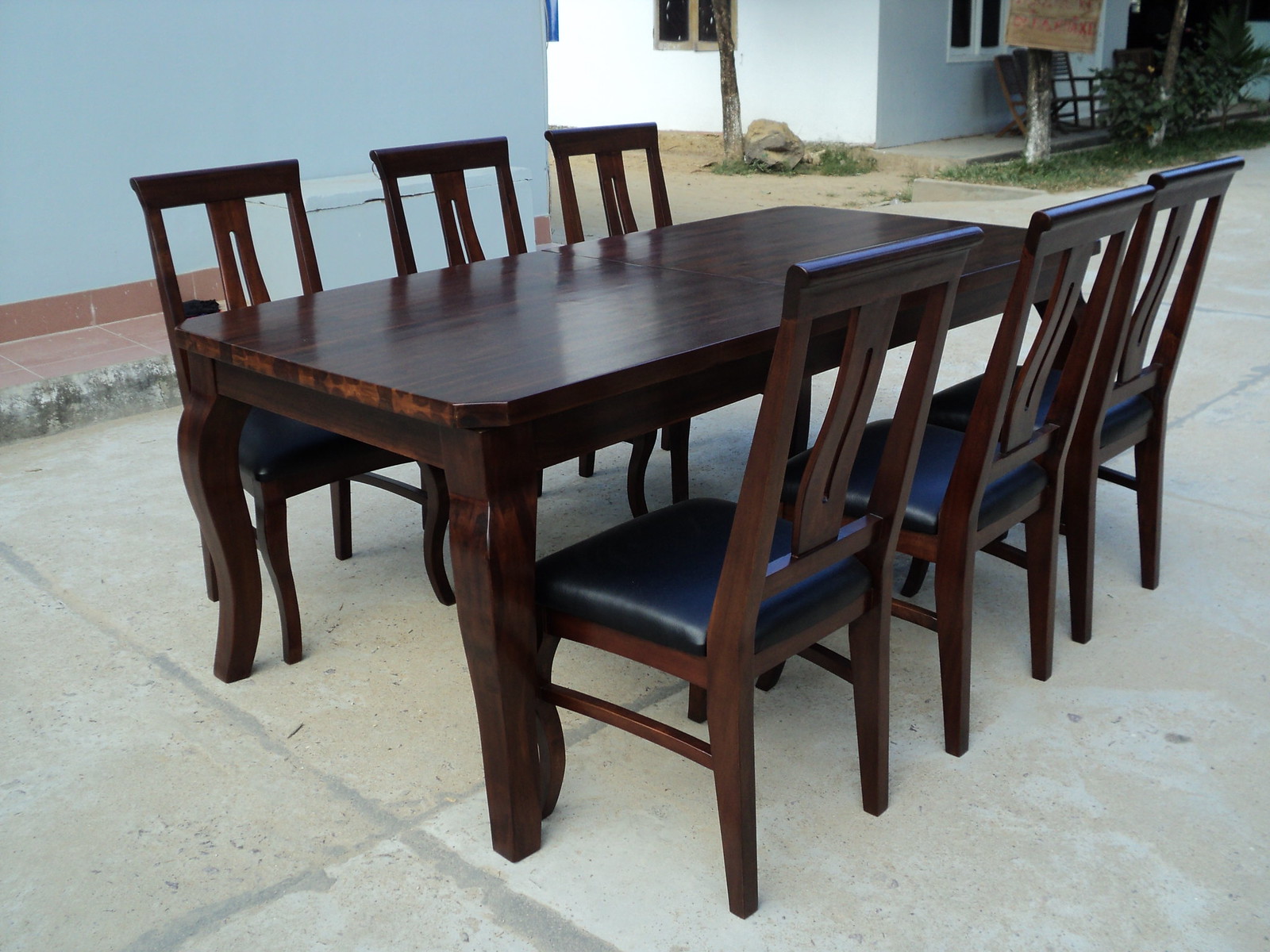The photograph captures an elegant dining setup placed temporarily on a concrete patio, suggestive of a backyard gathering or party. The focal point is a large, dark mahogany-stained wooden dining table accompanied by six matching chairs. The chairs, with legs and backs of the same rich, dark wood, feature cushioned seats covered in black vinyl or leather. Set against the backdrop of sky blue buildings, one of which features a window overlooking the scene, the visual is framed by elements like a grey concrete sidewalk, light grey street, and patches of greenery. The distinctive contrast between the luxurious indoor furniture and the outdoor setting underscores the temporary nature of this arrangement, enhancing the impression of a special occasion.